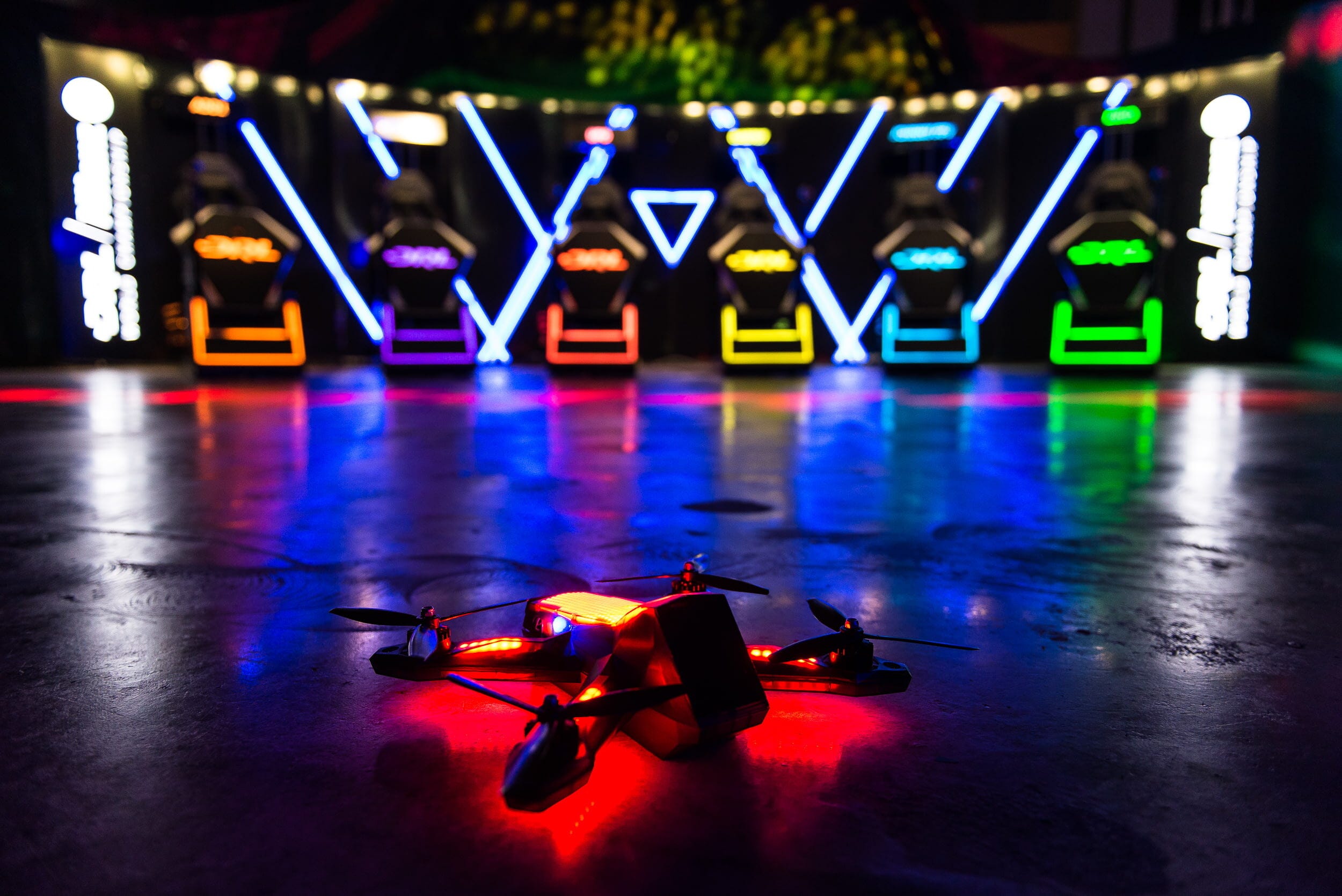A photograph taken at night reveals a vivid scene featuring a stationary drone in the foreground resting on polished, reflective concrete. The drone, adorned with red lighting, has four to five propellers and a phone-shaped section at its front. In the background, six ergonomically identical objects that resemble glowing professional gaming chairs, each illuminated by distinct neon colors—orange, purple, red, yellow, blue, and green—are arranged between white bars. The setting appears to be an arcade or game show area, with several screens positioned in front of the chairs. The surroundings, though mostly dark, hold sparkling elements on the ceiling, adding to the immersive atmosphere. A sign on the left side of the image remains unreadable due to the low lighting and focus.